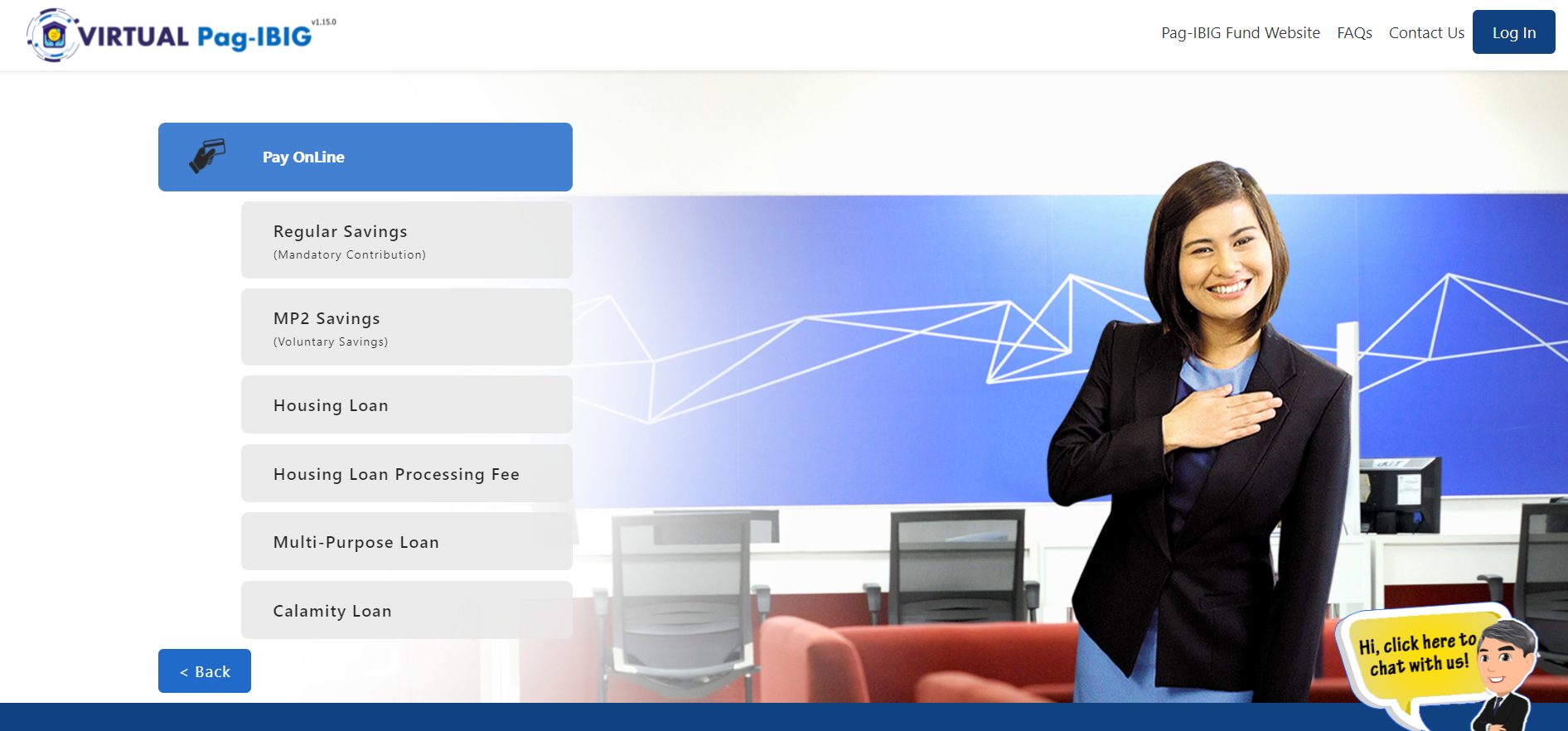The image displays a section of the PAG-IBIG Fund website, specifically highlighting the virtual PAG-IBIG online portal. The interface is organized with various savings and loan options neatly listed in a vertical menu on the left-hand side. At the top of this menu, within a blue panel, is the "Pay Online" heading. Below it, grey panels detail the available services: Regular Savings, MP2 Savings, Housing Loan, Housing Loan Processing Fee, Multi-Purpose Loan, and Calamity Loan. A blue "Back" button is situated below these options, providing easy navigation to the previous page.

In the top right corner of the screen, the PAG-IBIG Fund website is clearly identified, reinforcing the website's branding. Adjacent to this are links for "FAQs" and "Contact Us," both displayed in grey. A "Login" button is prominently positioned in the far top right corner for user access.

The central part of the screen features a splash image depicting an Asian woman, dressed in a blue outfit and black top, smiling warmly at the camera. She has her hand over her chest, possibly signifying a gesture of sincerity or welcome. Behind her are several chairs and what appears to be a large display screen. Complementing the friendly atmosphere, a cartoon character in the bottom right corner of the screen invites users to engage in a chat with a message that reads, "Hi, click here to chat with us."